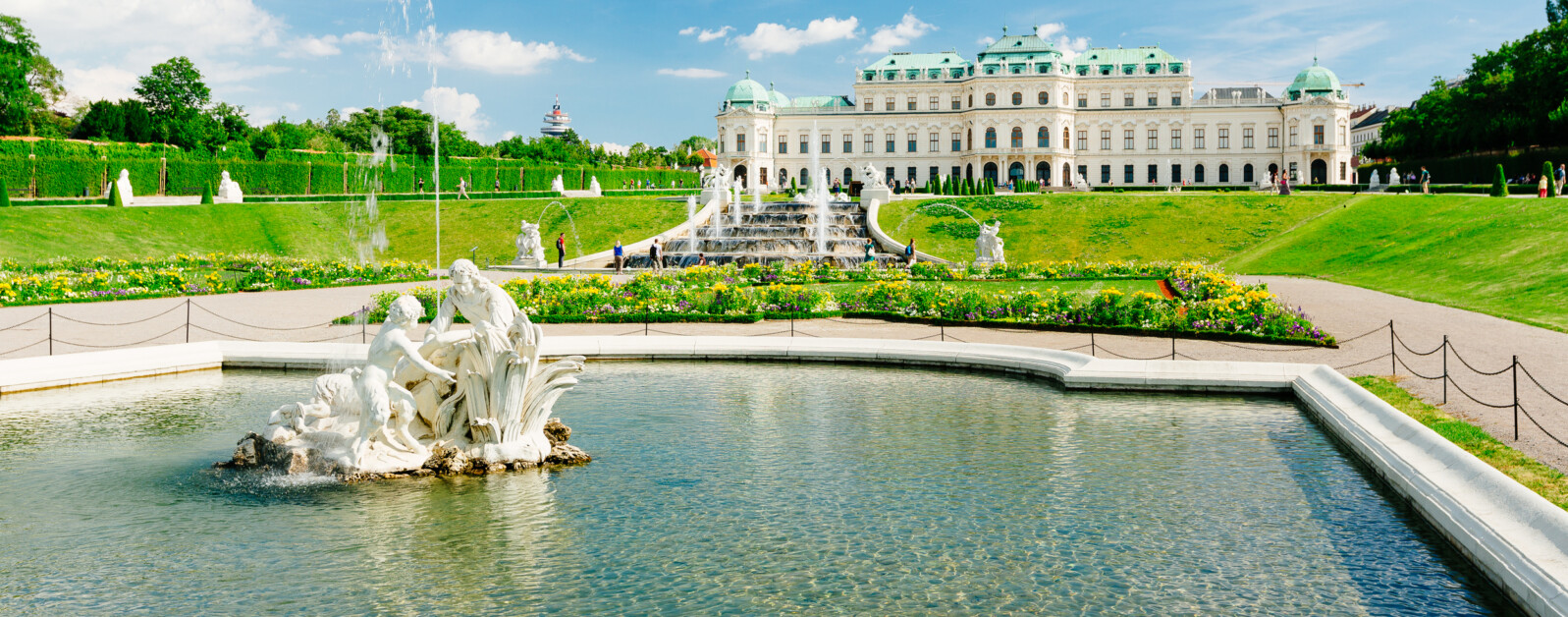In the foreground of this landscape-oriented photograph, a large fountain with a white border captures immediate attention. The fountain, adorned with a white statue of two people or children playing on rocks, has water sprouting elegantly between them. This fountain is situated in a pool of water that occupies the bottom half of the image. Flanking the pool, pathways with small black fences on either side converge in the distance, leading to a grand staircase. Beyond the pool and fountain area, lush green grass spreads out, interspersed with well-maintained small plants and flowers, primarily yellow with occasional purple blossoms.

People are seen leisurely strolling or standing within this verdant garden space. The scene is further enriched with the presence of hedges and trees towards the left. Beyond the garden, a majestic white building—reminiscent of a hotel or resort—stands proudly. This structure ascends three stories high, with an architectural middle section that slightly protrudes, flanked by symmetrical wings on either side, each with multiple rows of windows. The building's roofs are a soft green, contrasting with its pristine white walls. Trees are visible on both the right and left sides of the building, and a grassy hill extends into the background on the left. Above, the sky is a brilliant blue, flecked with white clouds, adding a serene backdrop to this picturesque setting.